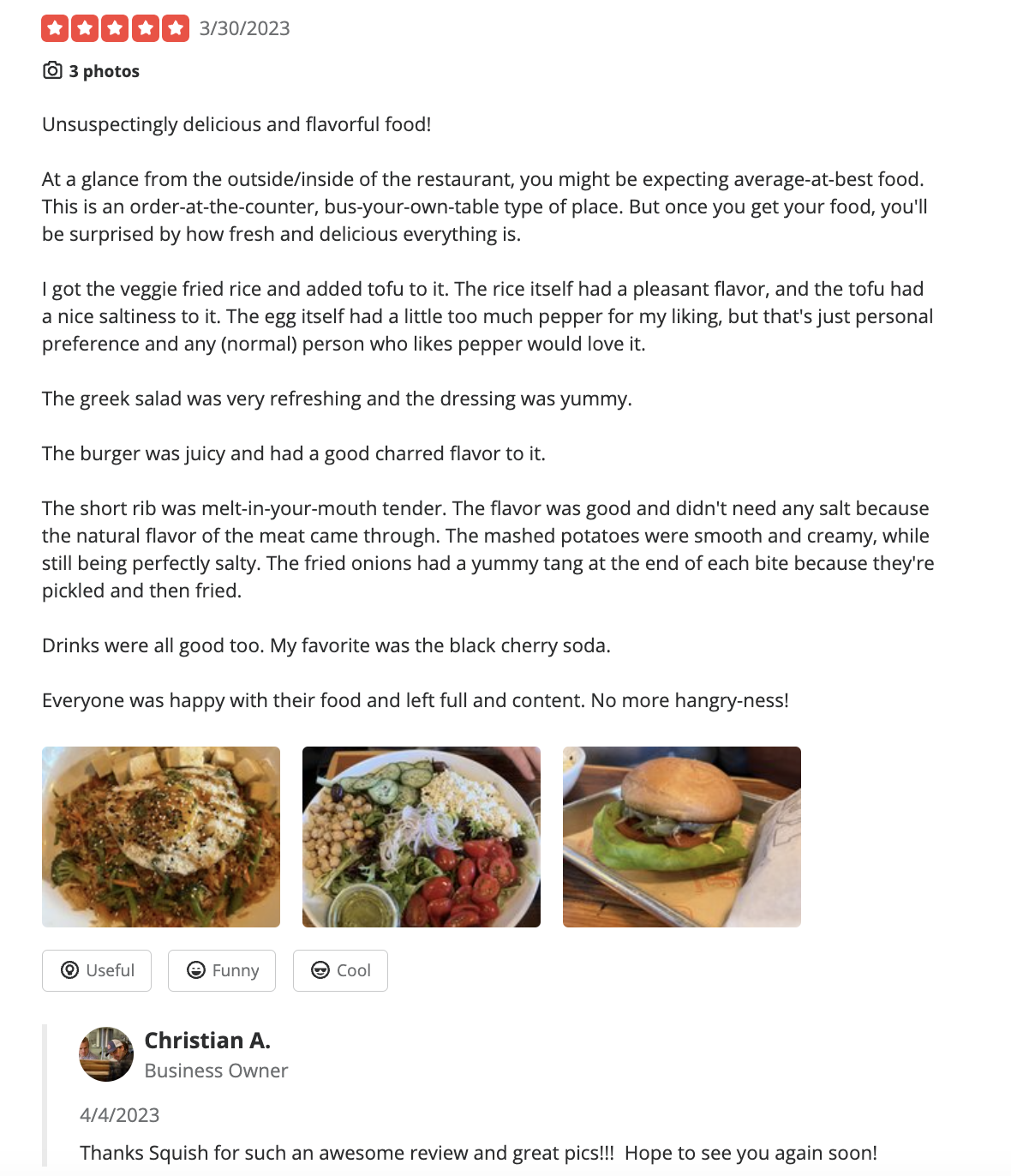Screenshot of a glowing five-star restaurant review dated March 30, 2023, showcasing exuberant praise for an unexpectedly delightful dining experience. The review features three tantalizing photos of the food: a meticulously seasoned egg dish, a refreshingly crisp Greek salad, and a succulent, char-flavored hamburger, positioned horizontally from left to right.

In the detailed review, the patron lauds the restaurant's "unsuspectingly delicious and flavorful food," noting that its modest exterior and order-at-the-counter setup belied the freshness and quality of the dishes. The reviewer highlights their veggie fried rice with added tofu, pointing out its pleasant flavor and perfectly salty tofu, although mentioning a personal preference against the peppery egg. They also rave about the Greek salad's refreshing nature and a delectable burger with juicy, charred meat. Standout dishes include melt-in-your-mouth tender short rib requiring no additional salt, creamy mashed potatoes, and tangy pickled fried onions. The reviewer also appreciates the delightful selection of beverages, highlighting the black cherry soda as a favorite. The overall sentiment is one of complete satisfaction, with everyone leaving content and no longer "hangry."

The review concludes with a response from Christian A., the business owner, dated April 4, 2023, expressing gratitude for the "awesome review and great pics" and extending a welcoming invitation for future visits.